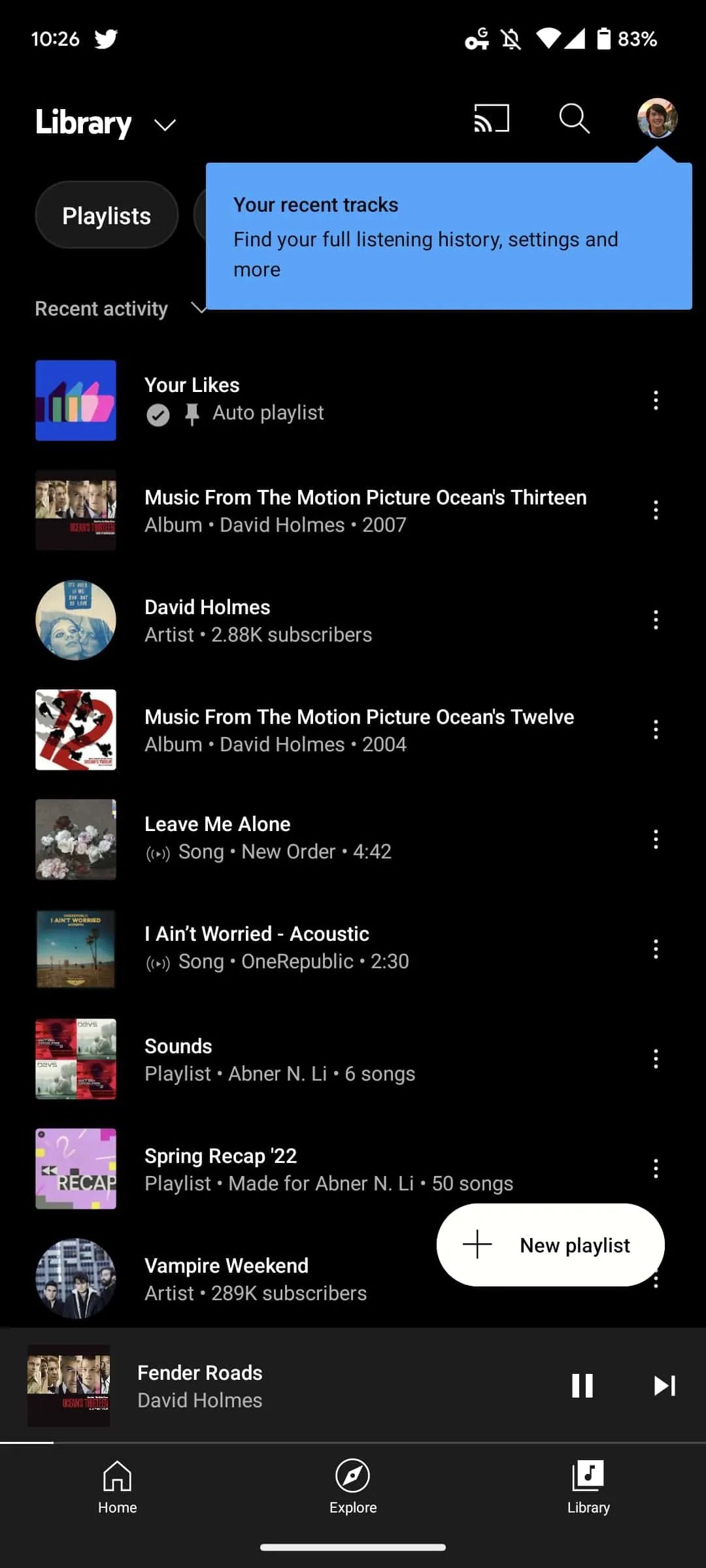This image depicts a detailed view of a music playlist interface on a black background. Starting from the top left, the screen displays the time "10:26" followed by the white Twitter bird logo. To the right of that, there's a key icon with the letter "G" on it, a crossed-out bell icon, full Wi-Fi signal, full cellular signal, and an 83% battery indicator.

On the left side of the screen, there's a "Library" label with a drop-down arrow beside it, followed by a screencast button, a search icon, and an avatar showing a Caucasian individual. Next to the avatar, a blue speech bubble points toward it, stating "Your recent tracks, find more, your full listening history settings, and more."

Adjacent to this, there's a "Playlist" label, followed by "Recent activity" in a drop-down menu format. Below this, there's a "Your likes" section, featuring an LGBTQ-themed thumbs-up square icon, labeled "Auto playlist" with a thumbtack and a gray check mark.

Further down, there is an image associated with the "Music from the Motion Picture Oceans 13" album by David Holmes, released in 2007. Below this image, there is another image under the "David Holmes" artist category, which notes "2.88K subscribers."

Next is a red and white image labeled "Music from the Motion Picture Oceans 12," followed by a gray background with the title "Leave Me Alone" by the band New Order. Another entry is an outdoor-themed image with a blue sky, labeled "I Ain't Worried" (acoustic) by OneRepublic.

Additionally, there's a playlist by Abner N.LI featuring six songs in red and gray, a pink square box labeled "Recap, Spring Recap 2022," which is a playlist made for Abner N, containing 50 songs. Lastly, there's an image of the band Vampire Weekend, noted as "2.89K subscribers" and featuring three Caucasian individuals.

At the bottom, the currently playing song or video is "Fender Roads" by David Holmes, featuring the same Oceans 13 imagery mentioned earlier. Playback controls include a pause button and a forward button. Below these controls, navigation options are displayed: a home button, an explore button, and a library button.